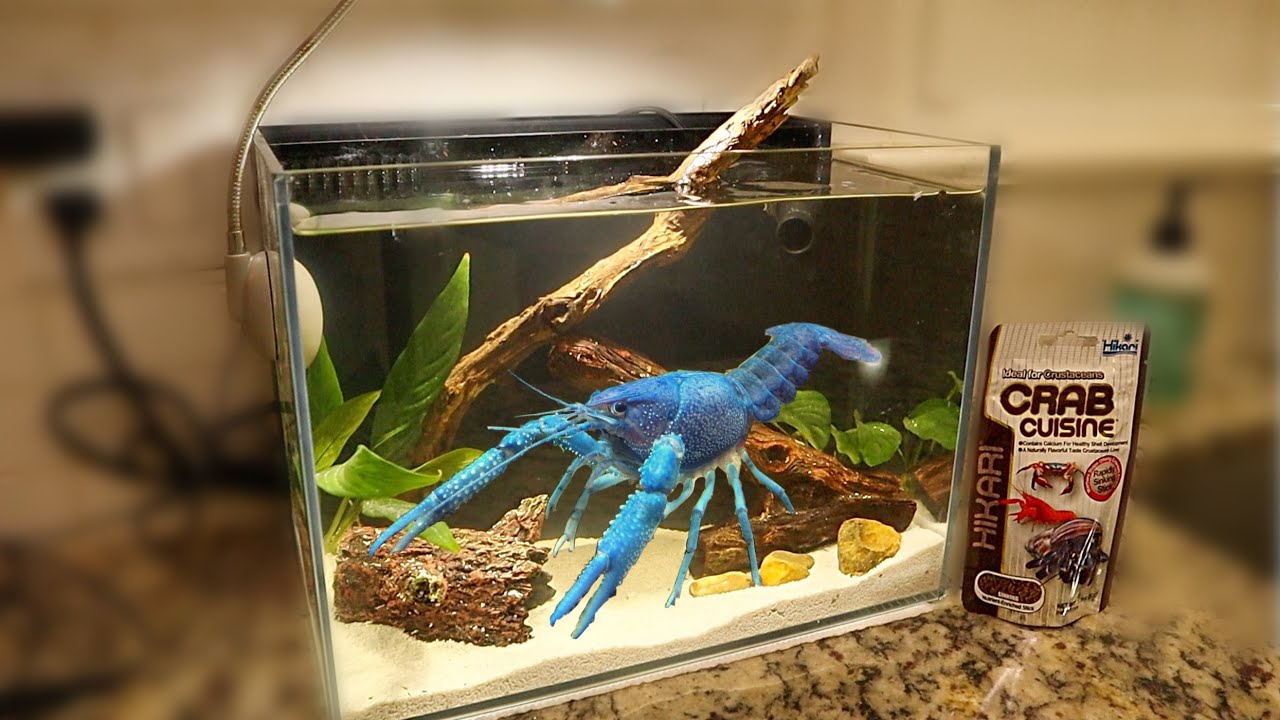The photo features a meticulously arranged aquarium positioned on a speckled granite countertop, characterized by its brown and beige marbling. Inside the aquarium, under an overhead light, a vibrant blue crustacean, possibly a highly edited blue lobster or crab, is seen facing left, appearing almost lifelike despite the Photoshop enhancements. The tank's decor includes driftwood, with a prominent piece extending from the bottom left to the upper right of the tank, occasionally breaking the water's surface, alongside some sand and greenery. Accompanying the aquarium, on the right-hand side of the countertop, is a small, unopened packet of Hikari Crab Cuisine, clearly labeled with an image of a crab. The background appears intentionally blurred, likely with a blurring tool, contrasting with the sharp focus on the aquarium setup, which is illuminated under indoor yellow lighting, suggesting the photo was taken inside a house or apartment.